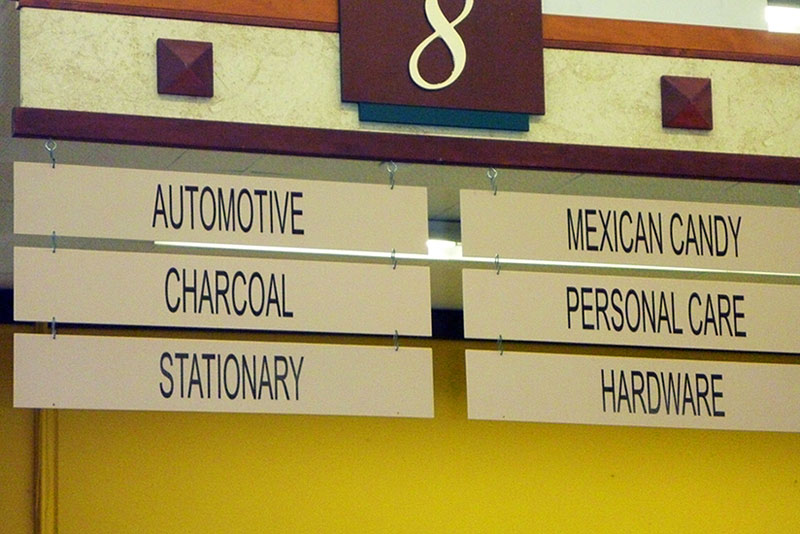In the image, we see aisle eight of a store, prominently marked with a white number "8" on a maroon background. This designation is part of a larger display featuring a marbled strip adorned with two decorative maroon squares and flanked by wooden borders. Suspended from this display are two hanging signs that catalog the items found in this aisle. The sign on the left lists "Automotive," "Charcoal," and "Stationary" in neatly divided sections. On the right, another sign segments "Mexican Candy," "Personal Care," and "Hardware." These signs are affixed with screws, emphasizing a well-organized layout. The backdrop is a warm yellow wall, complemented by a wooden border on the left-hand side, enhancing the inviting ambiance of this store aisle.